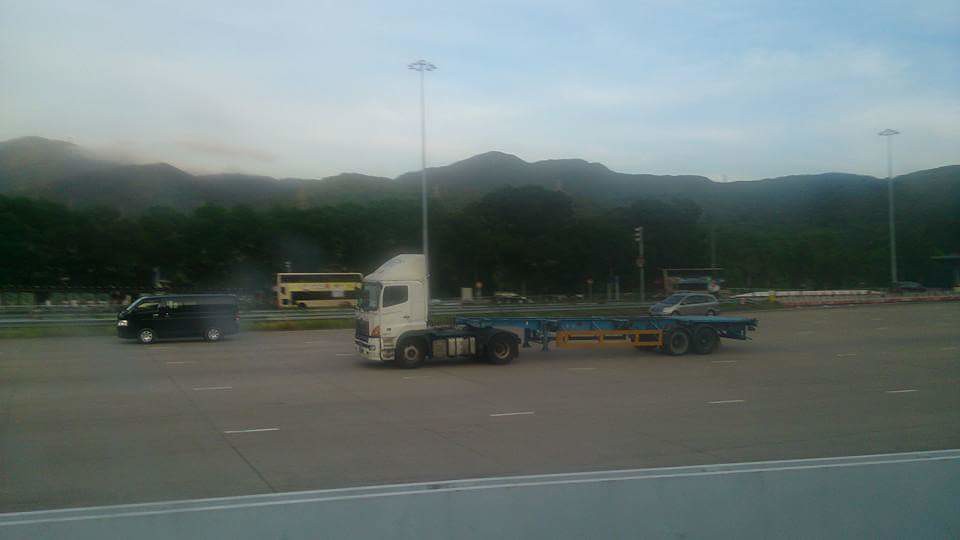This image captures a busy six-lane highway under a sunny blue sky, lightly dotted with clouds and fog around the mountainous background. The road stretches into the distance, flanked by towering lampposts and lane markings, indicative of a major interstate or motorway. To the right of the foreground, there's a detailed view of a white cab flatbed truck with a sloped cabin, hauling an empty cargo carrier. Nearby, a compact silver-gray hatchback and a blue-black van cruise along. Further back in the image, a vivid yellow double-decker bus with black windows can be seen. The image suggests early morning light, casting a gentle glow over the scene and the sparse tree line before the mountain range, which adds a serene touch to the bustle of highway traffic. Amidst the vehicles and natural scenery, there is a sense of motion and travel, captured through the lens from inside another vehicle, hence giving a partly blurred impression.